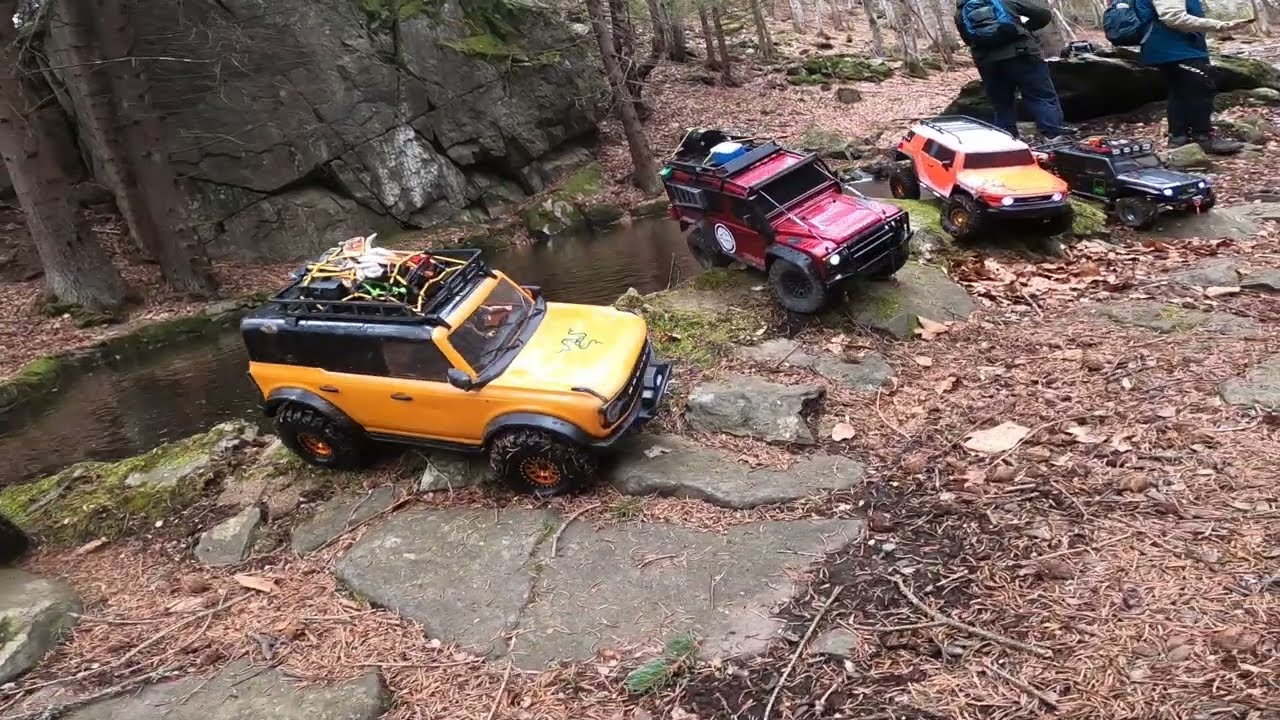The photo, taken outdoors, depicts four toy-sized jeeps positioned near the edge of a riverbank in a wooded area. The landscape is marked with dead or dying vegetation, hinting at a cold fall or winter day. Starting from the left, the jeeps' colors are yellow with big black tires, red with black, a predominantly orange jeep, and an all-black one. The third jeep in the lineup even features some white on its roof. Each vehicle also has cargo holds and baskets, with items secured by ropes.

In the top right corner of the image, two people are visible from the neck down. One wears a blue jacket with white arms and black jeans, while the other wears a gray jacket with blue jeans; both have blue backpacks. They stand amidst an array of brown leaves and are dressed for cooler weather, suggesting they might be preparing for a day of hiking. Behind the jeeps, a calm stream winds through the scene, flanked by large trees, a rock formation, and patches of green shrubs and algae.